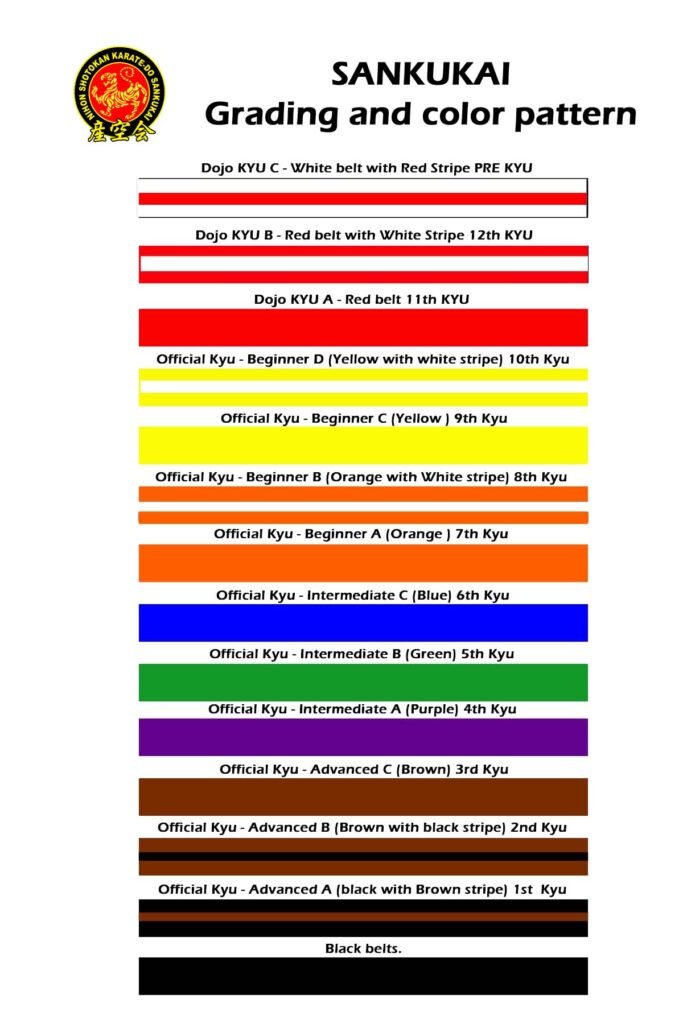The image is an infographic detailing the San Kukai karate belt grading and color pattern system. The title "San Kukai Grading and Color Pattern" is prominently displayed at the top in an italicized, sans-serif black font, in all capital letters. Below the title is the logo of a karate school, indicating that the infographic pertains to the dojo's belt ranking system.

The infographic visually represents the progression of belt colors from beginner to advanced levels, starting at the top with the lower rankings and moving downwards. The first belts listed are:

1. **Dojo KUC**: White belt with a red stripe (12th KYU)
2. **Dojo KUB**: Red belt with a white stripe (11th KYU)
3. **Dojo KYA**: Red belt (official KYU beginner)
4. **Yellow Belt with White Stripes**: (10th KYU official KYU Beginner D)
5. **Yellow Belt**: (9th KYU official KYU beginner C)
6. **Orange Belt with White Stripes**: (8th KYU)

This pattern continues, detailing each successive belt color and stripe variation, ultimately culminating at the bottom with the black belt, signifying the highest level. Each belt color and pattern is clearly labeled in a small black font similar to the title, ensuring clarity and consistency in the informational layout.

The infographic uses a combination of red, white, yellow, and orange colors to illustrate the various belt levels, emphasizing the progression and hierarchy inherent in the San Kukai belt grading system for karate practitioners.